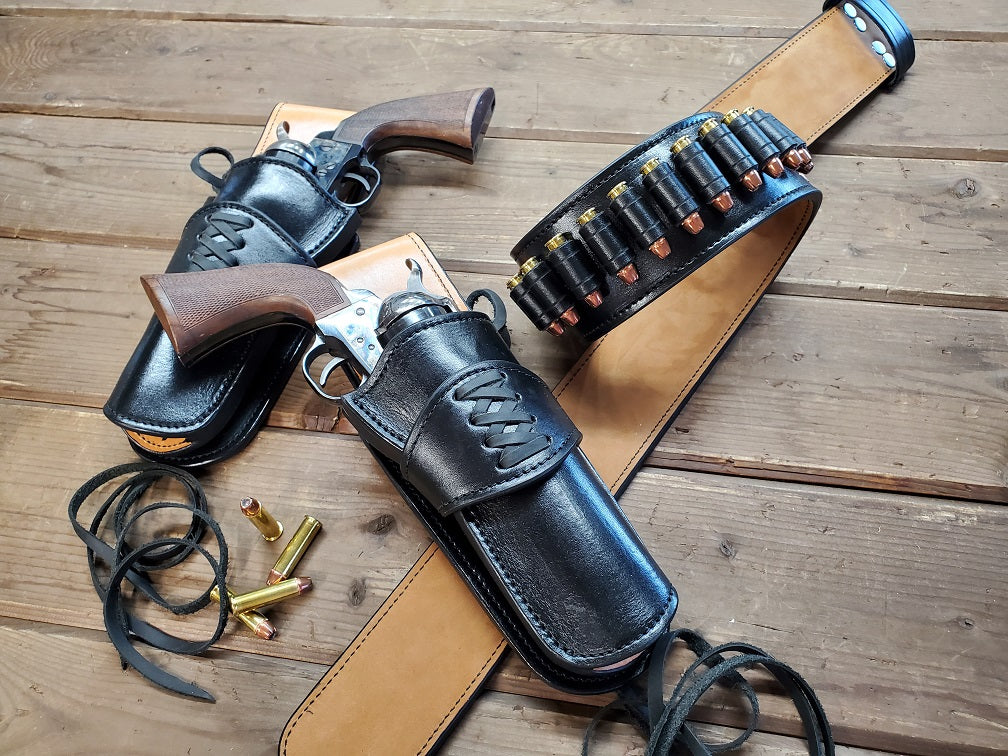The color photo captures a rustic scene set on a wooden floor made up of brown planks. Two old-style pistols with wooden handles and silver barrels rest inside thick black leather holsters, which feature lace-up details reminiscent of shoelaces. The holsters, detailed with stitching in the middle, are placed on a black leather gun belt. This belt, wrapped in a loop, showcases its tan interior and black exterior, adorned with numerous rounds of ammunition. The bullets, gold with copper tips, are fastened securely to the belt. Scattered between the two holstered guns are three additional bullets, each positioned differently—one stands upright, another lies slanted, and the third barely touches the others. A piece of string casually lies near the bottom of the guns, completing the meticulously detailed arrangement.